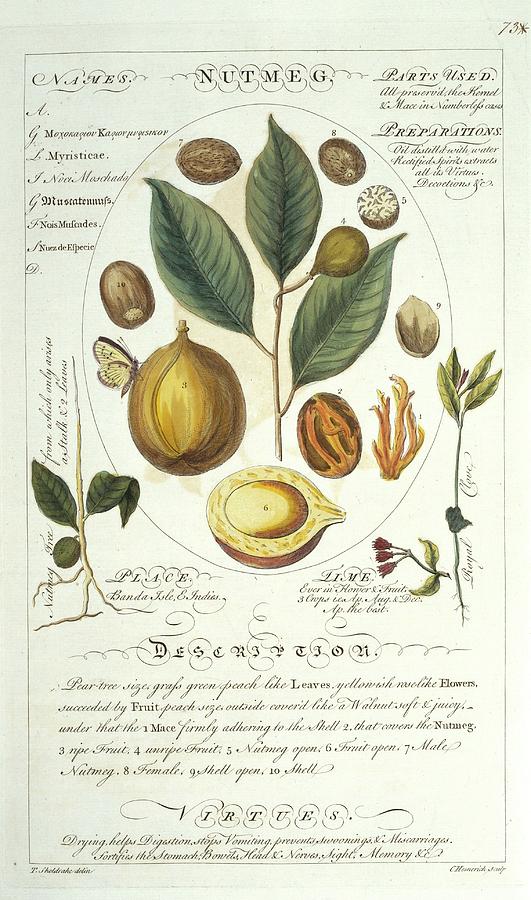This intricate, vintage botanical illustration represents Nutmeg (highlighted at the top with each letter circled) and is detailed and rich with color. The vertical image has a light-colored, slightly browned background that suggests an old page from a medicinal or plant book. A thin frame encircles the detailed drawings at its heart. Detailed illustrations showcase various parts of the nutmeg plant, including green, teardrop-shaped leaves attached to a brown stem, whole nutmeg seeds, nutmeg cut in half, revealing white and gray speckled interiors, and a close-up of the shell with a light yellowish hue. There's also an engaging depiction of a butterfly with yellowish wings and a purple body perched on a nutmeg seed, alongside a reddish bulb flower and more green leaves and stems.

Text elements dominate the top and bottom sections: at the top, “Nutmeg” is prominently displayed, and there's an index of parts used, preparations, and places where it grows, though the inscription is faint and cursive, making it tough to read. Adjacent to the botanical illustrations are various scientific names and possibly the virtues of nutmeg in black cursive text. Notably, the top right corner bears the number 73, paired with a small star symbol, adding to its antique feel. The entire composition gives an educational and artistic overview of the nutmeg, illustrating different parts and their uses, making it both an informative and visually appealing piece.